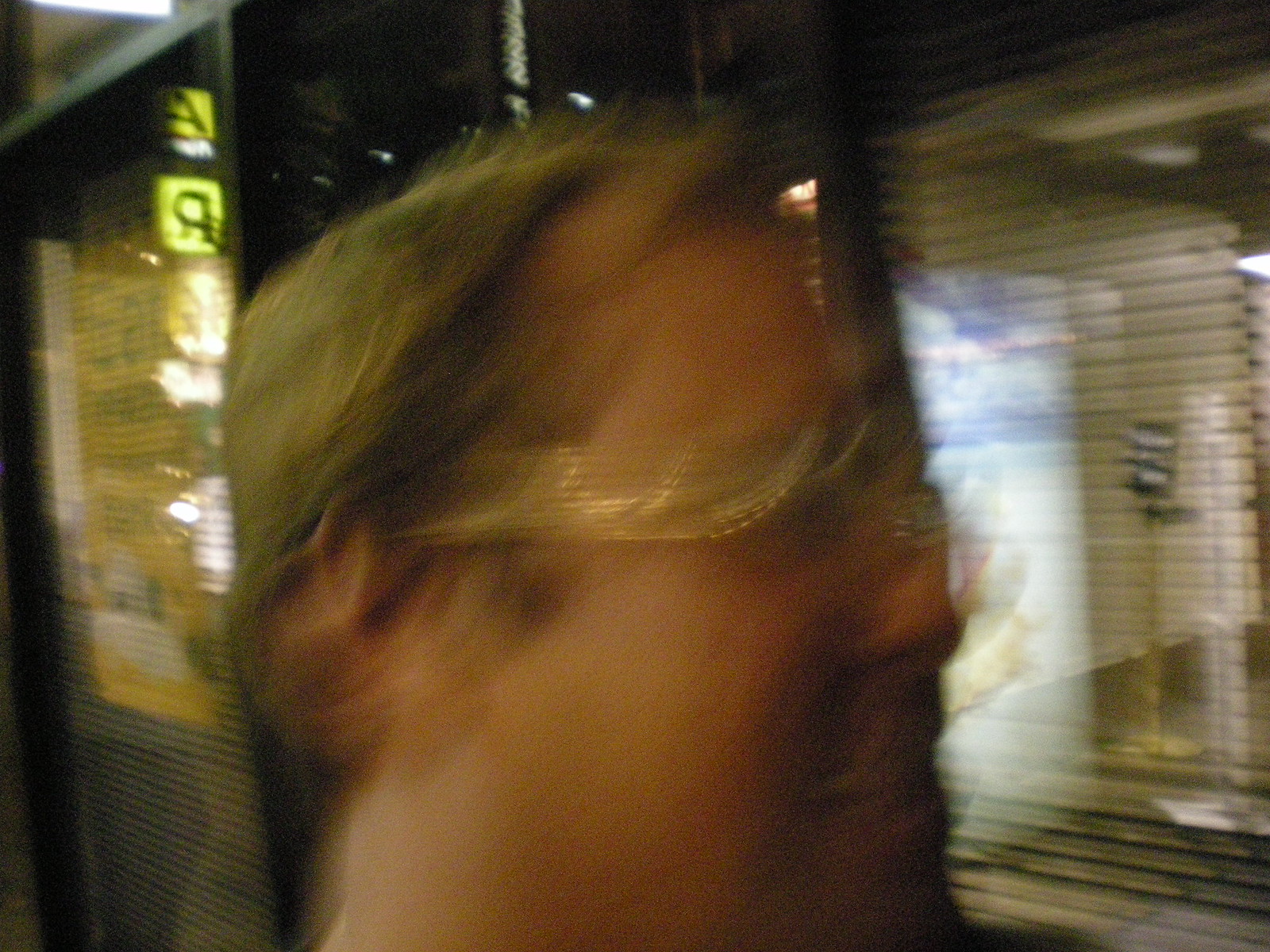This is a highly blurry and low-quality close-up image of the side of a man's head. The man, who has short blonde to brown hair, is wearing glasses, though most of his facial features, including his nose and eyes, are too blurry to distinguish clearly. He seems to be adorned with a gold headband that features a round piece or perhaps a feather in the center. He is facing towards the right side of the frame. The background is similarly blurred but reveals reflections of businesses through store or restaurant windows, indicating it's nighttime. Signs in the reflection mention "BAR" and "EAT." Blinds can be seen on the window to the right, and the lighting throughout the image is quite dim, adding to the photo's indistinct quality.